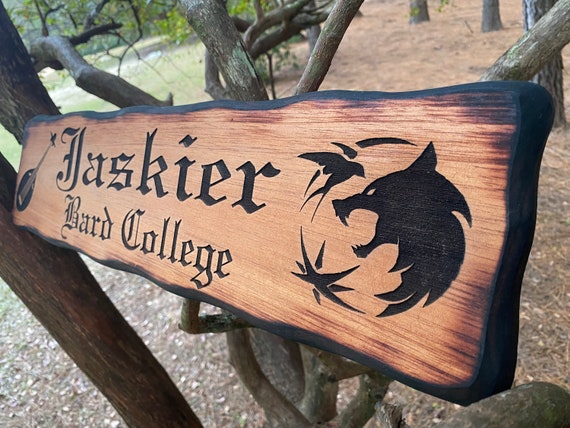The photograph captures an outdoor scene during the daytime featuring a wooden sign nestled on the gnarled branches of a barren tree. The sign, a long rectangular plank, appears to have been artistically burnt along its edges, giving it a distinctive dark border. Positioned amid twisting branches, the reddish-hued wood measures around 4 inches wide and varies in height, from 2 inches on the right down to 1 inch on the left.

On the leftmost part of the sign, there's an engraving of a stringed instrument, likely a mandolin or banjo. In the center, the inscription "Jaskier Bard College" is elegantly written, reminiscent of the New York Times font. To the right, there's a detailed emblem – a circular design featuring a wolf’s head with fangs bared. This emblem includes a dove flying above the wolf, seamlessly completing the circle.

The scene is set against a forest floor strewn with brown leaves, while some trees visible in the background retain a few green leaves, enhancing the natural outdoor ambiance.